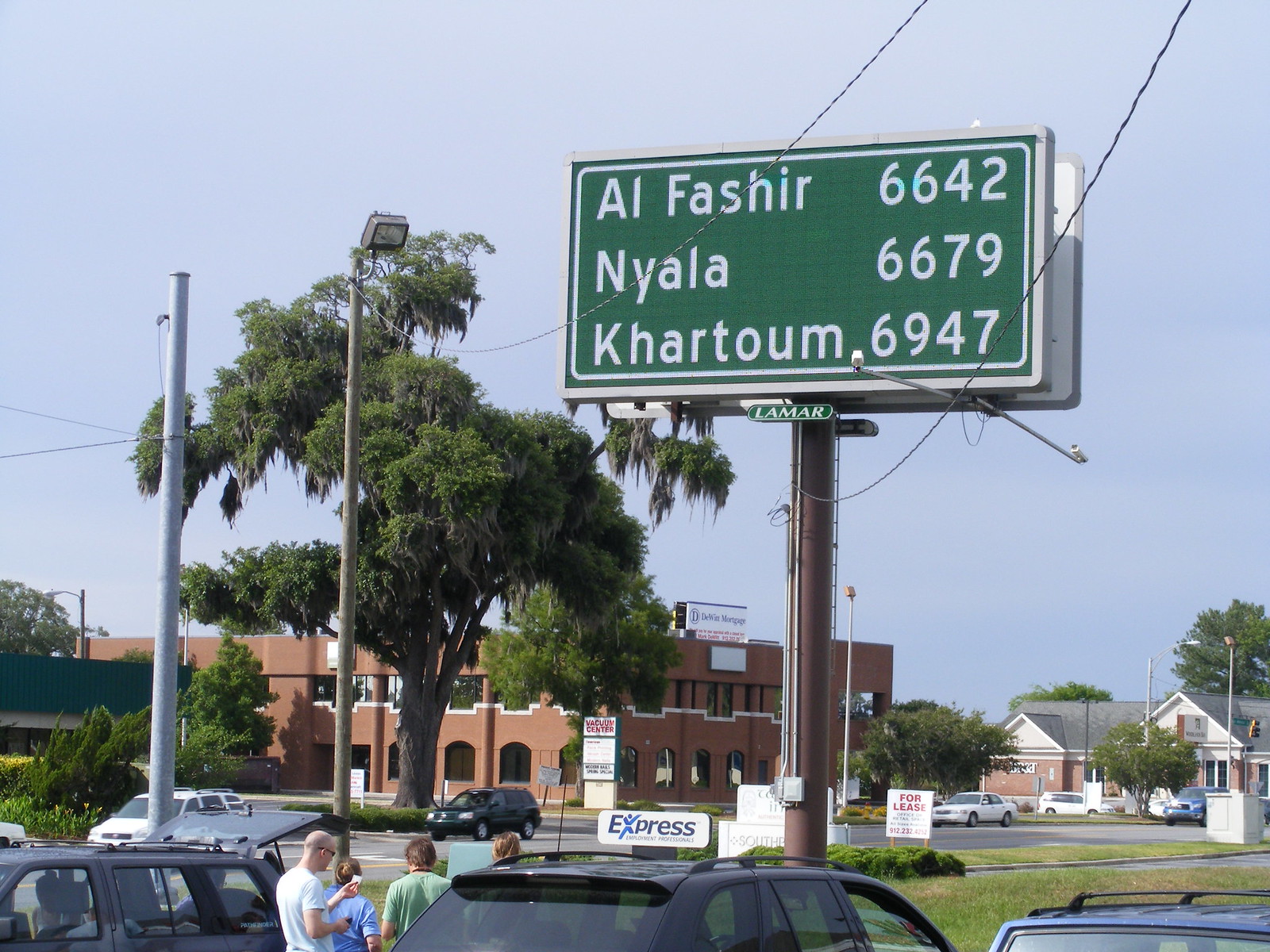This image captures a vibrant neighborhood scene on a clear, blue day. Dominating the foreground is a large green road sign displaying the distances to Al-Fashir (6642 km), Niyala (6679 km), and Khartoum (6947 km). Scattered around the vicinity are other signs, including one labeled "express" and another "release."

In the background, a two-story red building with distinct Moroccan-inspired architecture stands out, adding a touch of cultural flair to the neighborhood. Nearby, a house with a gray roof and white exterior complements the scene, contrasting against the lush greenery.

A tall tree with hanging green leaves adds a touch of nature, and a series of telephone poles extend into the distance, hinting at the neighborhood's layout. Various cars are parked in the foreground, including a family standing beside one vehicle. Among them, a man in a white shirt appears to be looking at something, while other family members in blue and green shirts stand nearby, engrossed in their surroundings.

The detailed elements in this image collectively paint a lively picture of everyday life in this neighborhood.